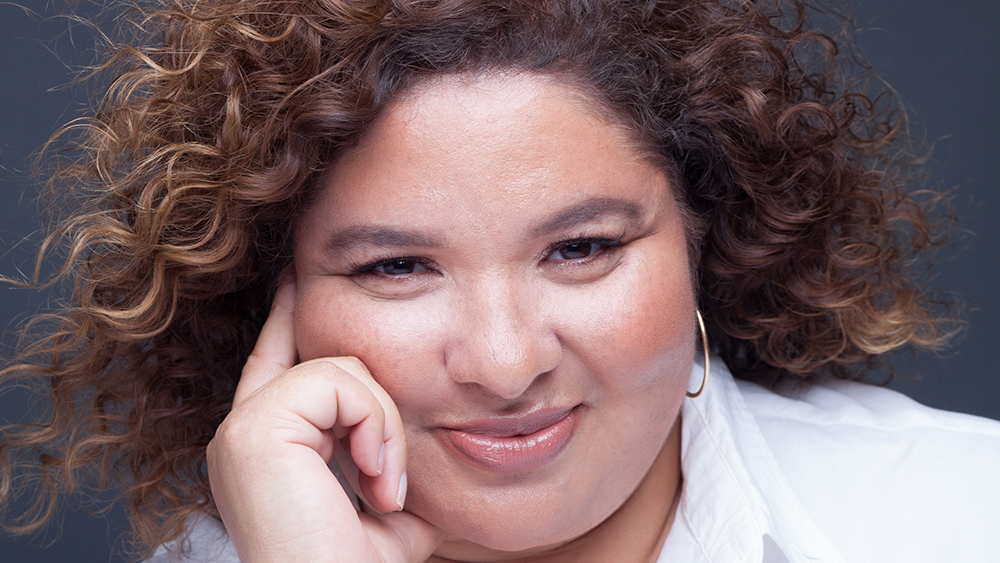This is a wide-format headshot of a smiling woman with her mouth closed. She has a round face with light brown skin, and her dark brown, curly hair reaches about chin to neck length, featuring some highlighted golden strands that add volume. Her expression includes a slight squint which accentuates her full lips. She is wearing a white collared shirt and gold hoop earrings—one of which is slightly visible on her left ear. The background is a subdued, dusky blue or blue-gray color, focusing attention on her expressive face and understated elegance.